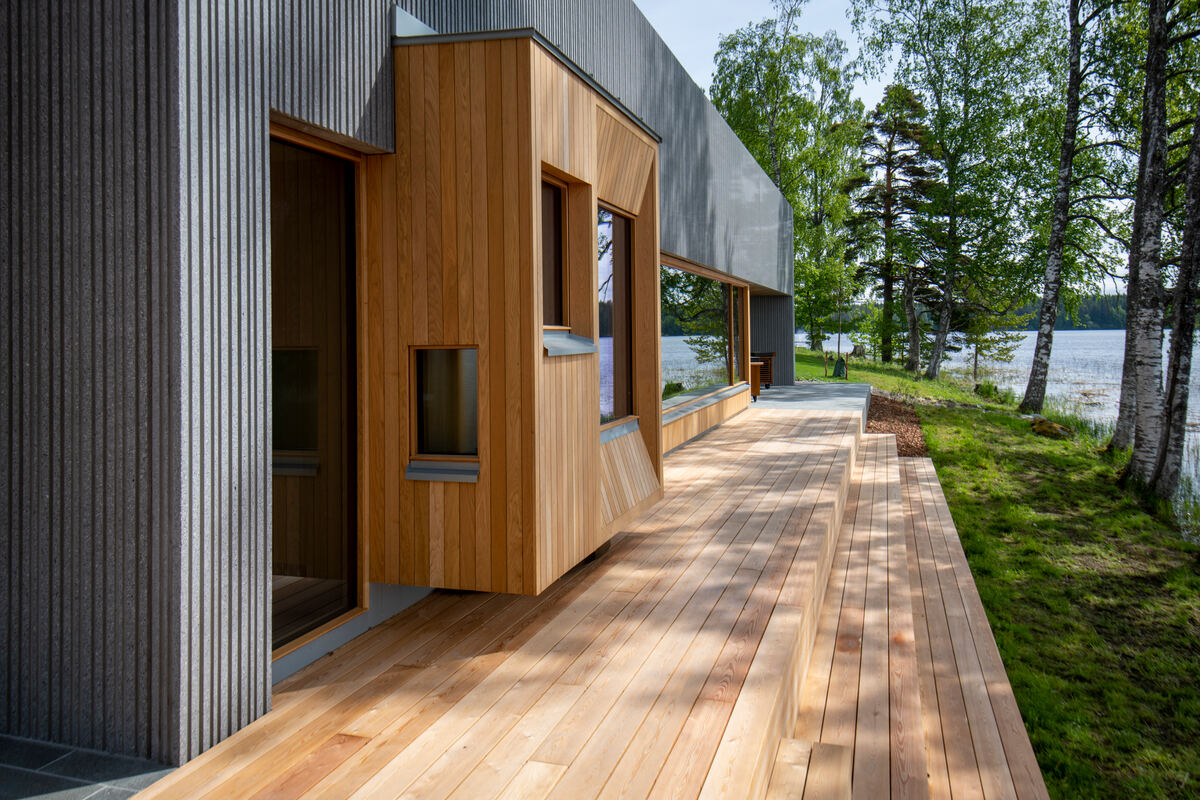This professional photograph captures a striking, modern, minimalistic lakeside building, partially constructed with unfinished bare wood. The building, extending vertically downwards in the frame, features a top section in gray and a middle section of bare, untreated wood. A notable detail is the wooden staircase and patio at the front of the building, revealing raw wood steps that emphasize the structure's unfinished aesthetic. The building is adorned with large windows, including a prominent long one on the right side that allows a glimpse into the dark interior.

Surrounding the building is a lush, grassy area with several tall trees that have green leaves, contributing to a serene, natural setting. In the background, a shimmering lake can be seen, reinforcing the structure's lakeside location. The scene is bathed in sunlight, which filters through the trees and casts intricate patterns, silhouettes, and shadows onto the building, adding to the picturesque quality of the photograph. The bright blue sky further enhances the tranquil, pristine atmosphere of this architecturally striking lakeside retreat.